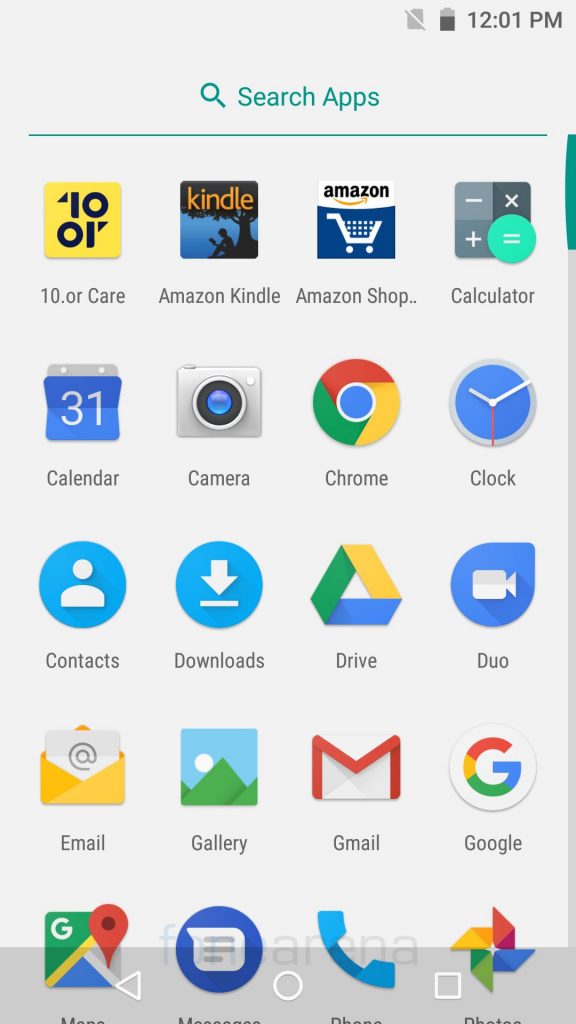The image depicts a smartphone screen showcasing an application interface. Dominating the top portion is a prominent, teal blue search bar featuring a magnifying glass icon and labeled "Search apps." Below this bar, a teal blue line indicates the input field for typing search queries. 

The screen displays a vertically scrollable list of apps set against a white background. The app icons appear in their typical, colorful designs. The highlighted apps from top to bottom include: 

- 10.org Care
- Amazon Kindle
- Amazon Shopping
- Calculator
- Calendar
- Camera
- Chrome
- Clock
- Contacts
- Downloads
- Google Drive
- Google Duo
- Email
- Gallery
- Gmail
- Google
- Google Maps
- Messages
- Phone
- Photos

At the very bottom of the screen, partially visible text suggests additional apps that are cut off from view. The bottom navigation bar features three essential icons: a back arrow, a home button, and a button for accessing recently opened apps. Adjacent to the app list, a teal blue scrollbar, matching the search bar's color, serves as an indicator of the extensive scrollable content, currently positioned at the top.